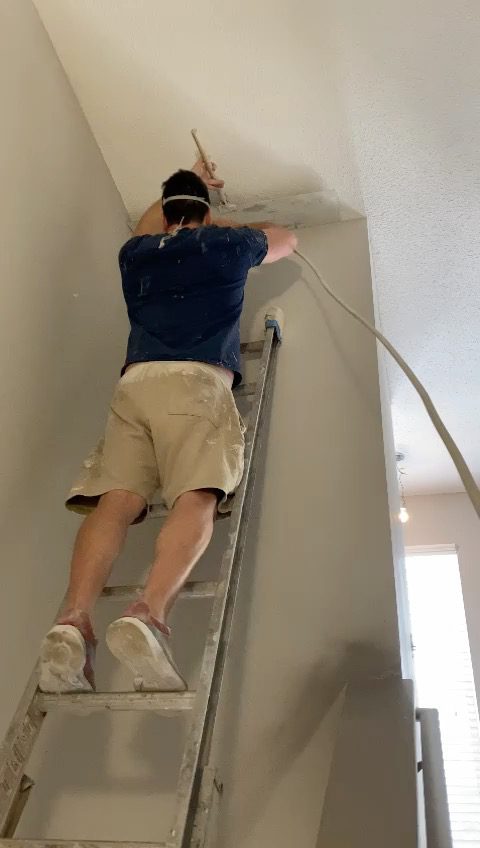In this vertical photograph, a man is seen working indoors while standing on the second step of a metal ladder, which is propped flat against a beige wall. The ladder is fitted with protective pads at the top to prevent damage to the wall's surface. Captured from a low angle, the image showcases the man's back as he attends to a task at the seam between the ceiling and the top of the wall, possibly painting. He is dressed in a dark blue t-shirt and beige shorts, both speckled with paint, and his sneakers also display paint marks on the soles. A long cord drapes from under his right elbow towards the center right of the image. The background reveals an adjoining room with similar beige walls, featuring a hanging light bulb without a fixture and a tall window with a shade, through which abundant sunlight streams in. A banister occupies the lower right-hand corner, adding depth to the scene. The man's shadow casts prominently on the wall below him, adding a dynamic element to the composition.